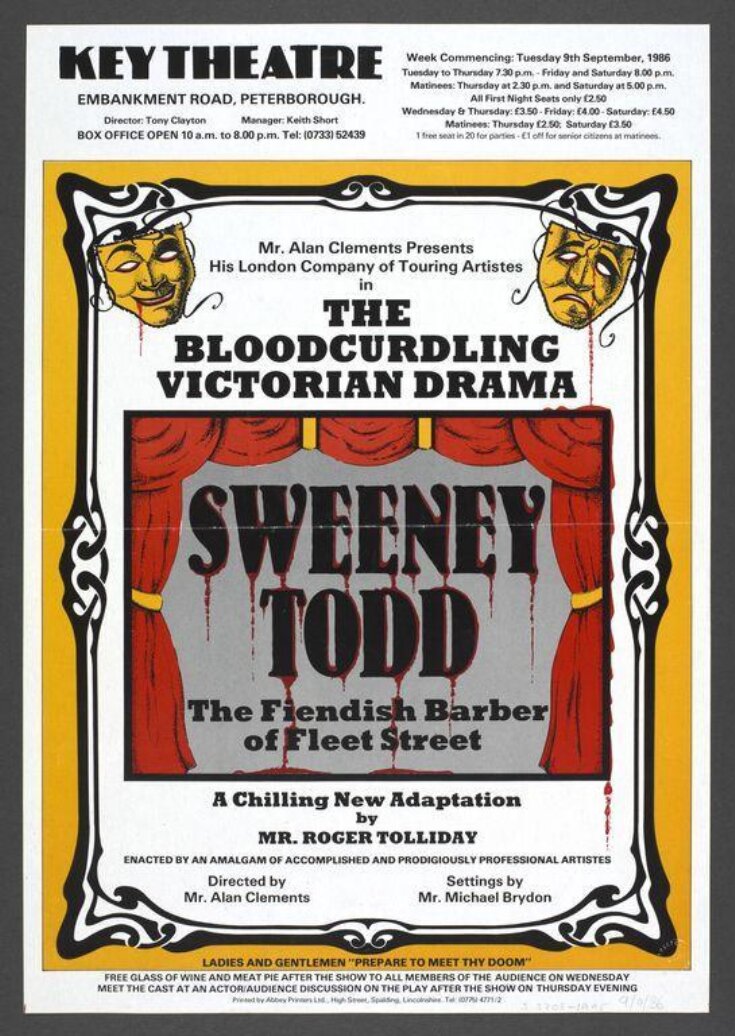This image features a detailed poster for a theatrical production. At the top left, it displays "Key Theatre, Embankment Road, Peterborough," and includes essential details such as the box office hours (10 a.m. to 8 p.m.) and the telephone number (0733-52439). The poster lists ticket prices and schedules: week commencing Tuesday, 9 September 1986, with performances on Tuesday and Thursday at 7:30 p.m., Friday and Saturday at 8 p.m., and matinees on Thursday at 2:30 p.m. and Saturday at 5 p.m. Ticket pricing varies, with all first night seats at £2.50.

In the middle of the poster, there is a smaller image framed by striking red curtains and topped with theatrical masks: one smiling and one sad. The centerpiece features blood dripping from the title "Sweeney Todd, The Fiendish Barber of Fleet Street." This blood-curdling Victorian drama is presented by Mr. Alan Clements with his London company of touring artists. Below, it notes the chilling new adaptation by Mr. Roger Soliday, alongside various contributors' names. Additionally, it mentions special offers such as one free seat for every twenty for parties and a senior citizen discount for matinees.